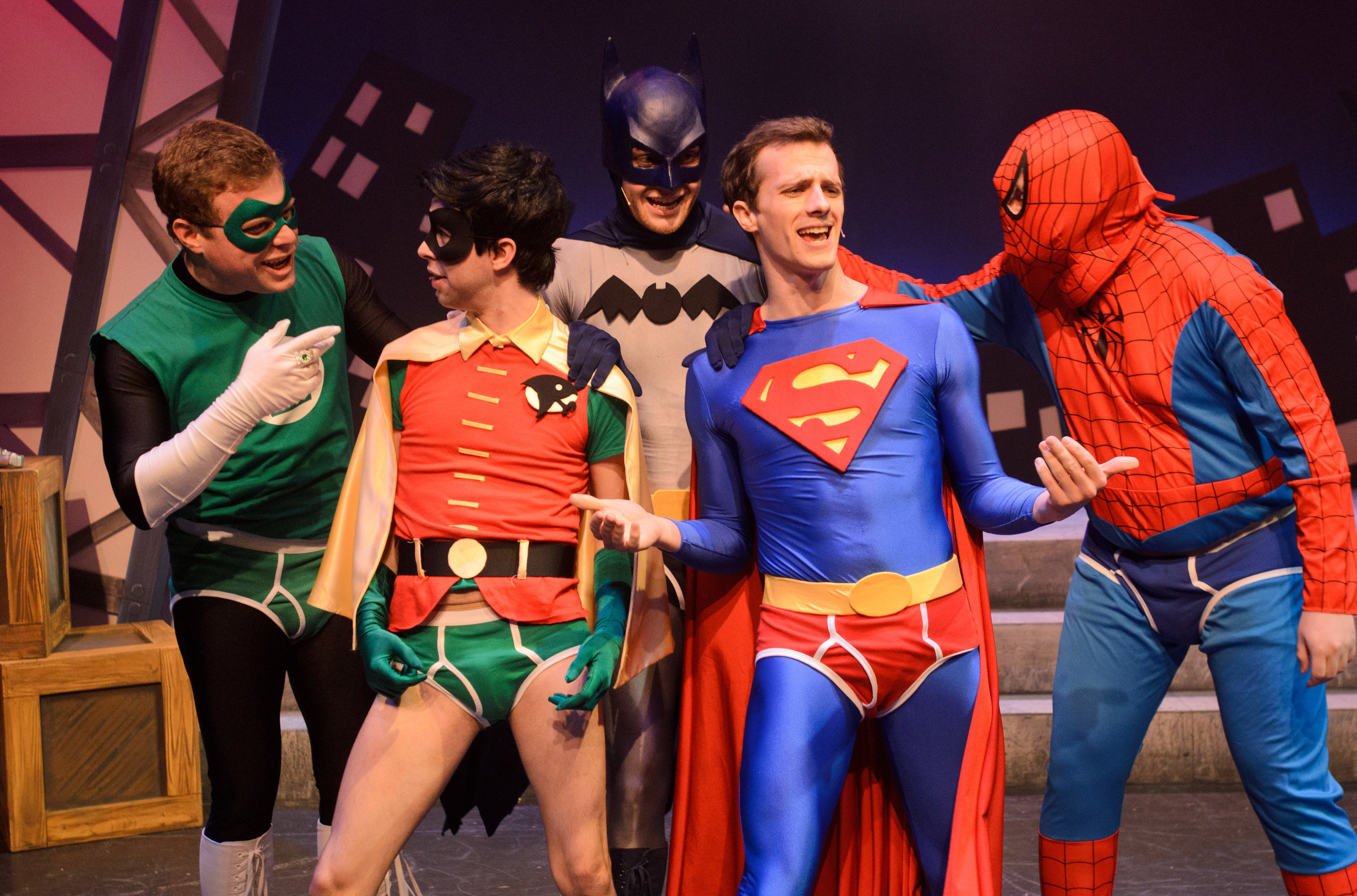The image portrays five adult men on a stage, each dressed in various superhero costumes, participating in what appears to be a comedic play or sketch show. On the far left, a man with light brown hair is dressed as Green Lantern, wearing a green and black costume with green and white underwear briefs over it, white boots, and a green mask. Next to him stands a man in green and white underwear with a red vest, yellow cape, green sleeves, green gloves, and a black mask, resembling Robin. In the center, a man dressed as Batman sports a green costume with a black cape and mask, featuring a black bat symbol on his chest. To his right, another man is clad in a bright blue costume with red underwear, a yellow belt, and an 'S' on his chest, portraying Superman. The far-right figure is dressed as Spider-Man in a costume with blue and white briefs, blue pants, red boots with black web patterns, and a matching red and blue shirt and mask. The stage is adorned with stylized crates, buildings, and stairs as a backdrop. The men are all pointing at each other, laughing, and smiling, indicating a lively and humorous atmosphere, with their homemade-looking costumes adding to the comedic effect.